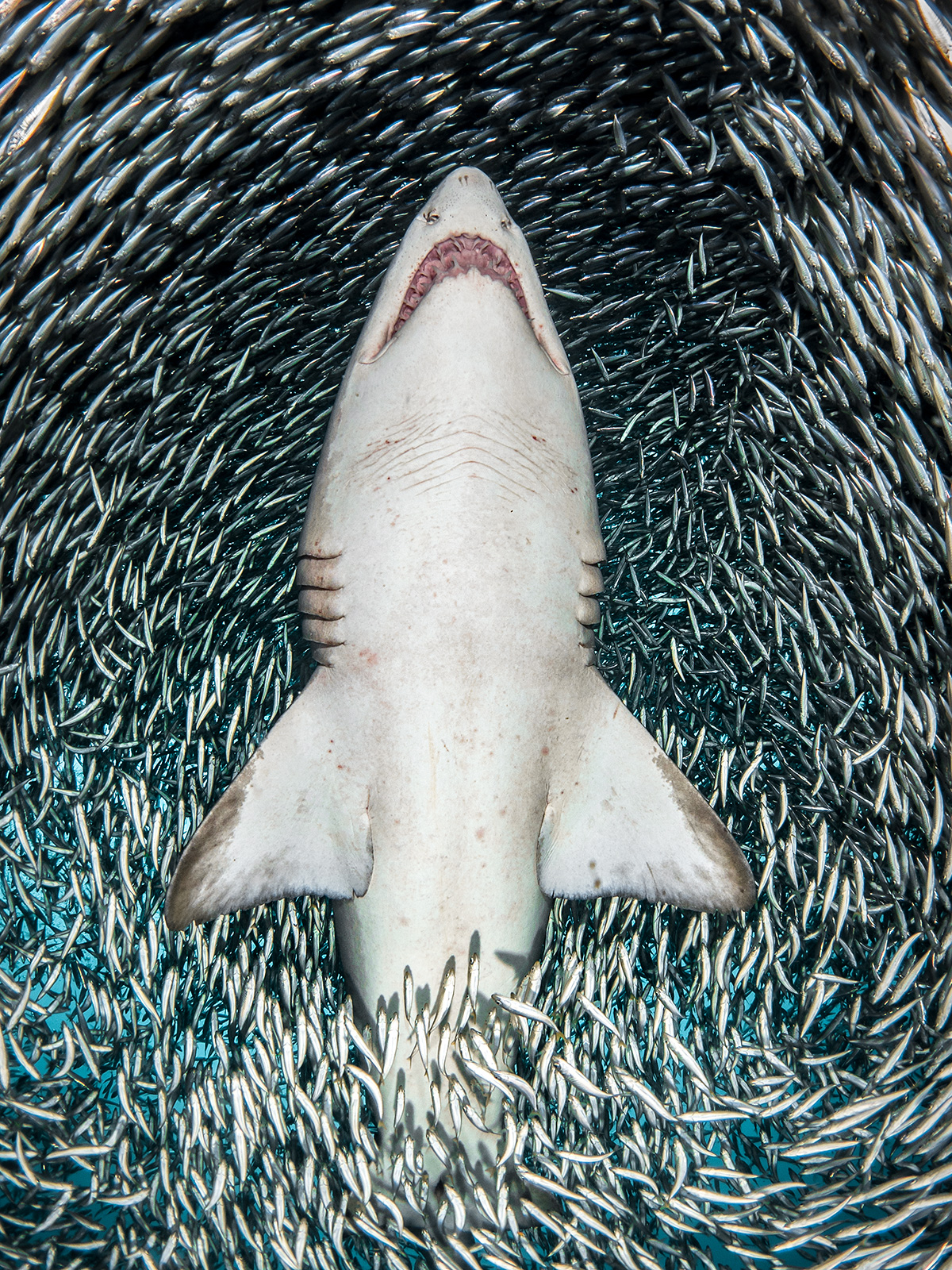The image is a striking and digitally altered underwater photograph of a shark viewed from below, showcasing its journey through a swirling vortex of tiny, silver fish. The shark, with its distinct white belly and dark-tipped fins, has its mouth slightly open and gills visible as it pushes upwards through the chaotic school of fish. These small fish, scattered like a thousand sardines or anchovies, create a mesmerizing silver-and-black tapestry around the shark, enhancing the sense of motion and dispersal as they attempt to evade the predator. The grayish silver hues of the fish contrast with the shark's more solid coloration, emphasizing the dynamic interaction within the ocean's depths.